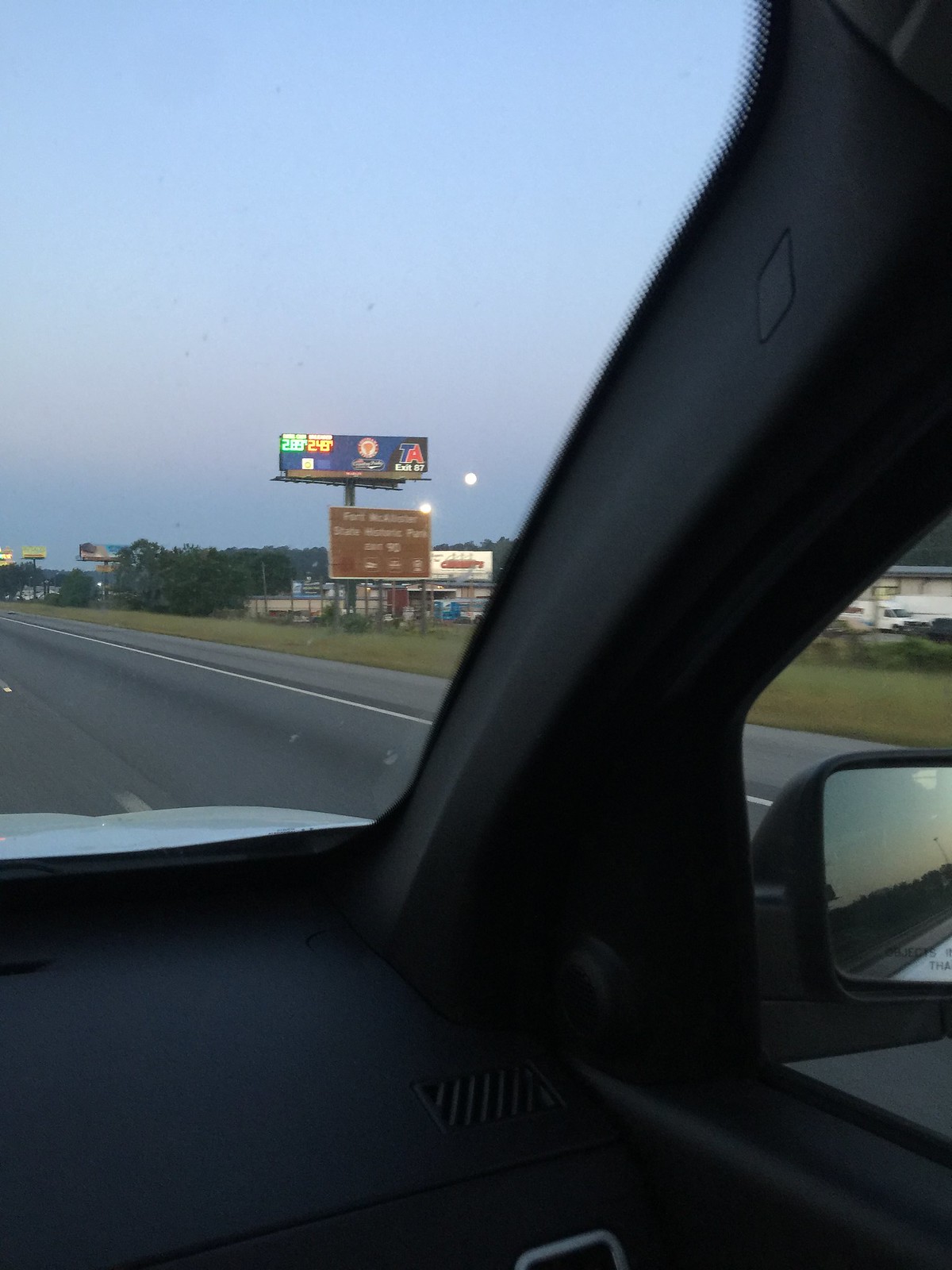The photograph appears to be taken from the passenger seat of a car, capturing a slice of life on the road. The vantage point from the side window gives a partial view of the side mirror and reflects a serene late evening sky. To the left, you can see the distant, calming shade of dusk beginning to envelop the horizon. There's a prominent brown sign indicating "Fort McAllister State Historic Park" with an exit number 90. Above it, a billboard advertises the TA travel center at exit 87, listing gas prices at $2.89 for regular and $2.49 for diesel. The foreground through the windshield reveals a collage of everyday roadside elements: a grassy embankment edged with trees, various buildings, and several vehicles adding dynamism to the still image. The sky, not fully dark but advancing towards twilight, hints at the impending evening with a touch of both the sun and possibly the moon faintly visible at a distance. Further down the road, other billboards pepper the side of the street, extending the vista into the fading light.